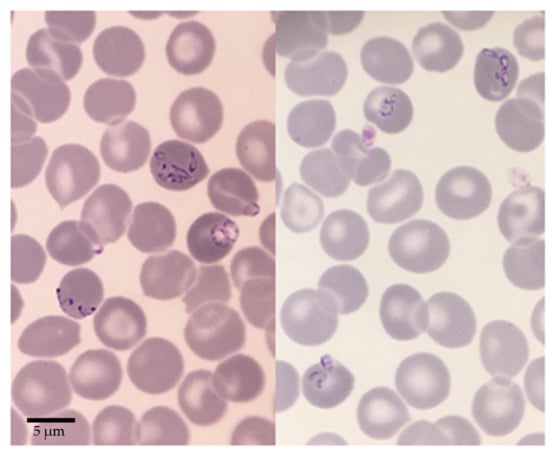The image under discussion appears to be a split-screen view of cell specimens captured under a microscope, with two side-by-side panels showing similar objects. The left panel displays what seems to be a cluster of cell organisms resembling small grapes or conkers, set against a light pink to orangish background. Some of these cells feature small purple or black dots, possibly indicating some sort of infection or abnormal growth. The right panel mirrors this layout but has a cream-colored, washed-out backdrop with the cells appearing more grayish. There is a slightly different arrangement of the cells between the two panels. In both images, a notation "5UM" with a measurement bar is visible, suggesting a scale of 5 micrometers. This annotation, located at the bottom left, is critical for understanding the size of these cellular structures.